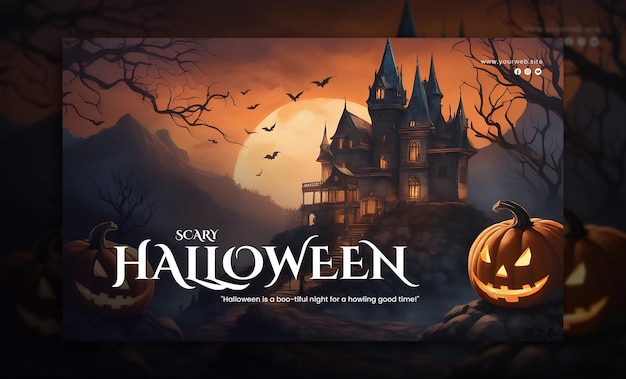This detailed and cleaned-up caption enhances the description of the image:

The image appears to be a screenshot from a laptop, displayed in landscape mode. Central to the image is a card that closely mirrors the background, effectively making the card a close-up representation of the backdrop. The card's main focus is an image featuring the text at the bottom: "Scary Halloween. Halloween is a boo-tiful night for a howling good time." 

In the bottom right-hand corner of the inner image, there is a jack-o'-lantern with glowing yellow eyes, a nose, and a serrated mouth, all illuminated by a candle inside the pumpkin. The pumpkin's stem is shown curved. 

The haunting backdrop features a menacing mansion with multiple rows, cupolas, and floors, adding an eerie atmosphere. To the left of the mansion, bats are silhouetted against a massive setting sun or rising moon, casting an orange and dark glow across the sky. 

In the upper left-hand corner of the image, a dead tree stretches its barren branches. Another jack-o'-lantern resides in the bottom right-hand corner. The upper right-hand corner of the image displays the text "www.yourweb.site" followed by the Facebook logo, suggesting that this is an advertisement to create your own website.